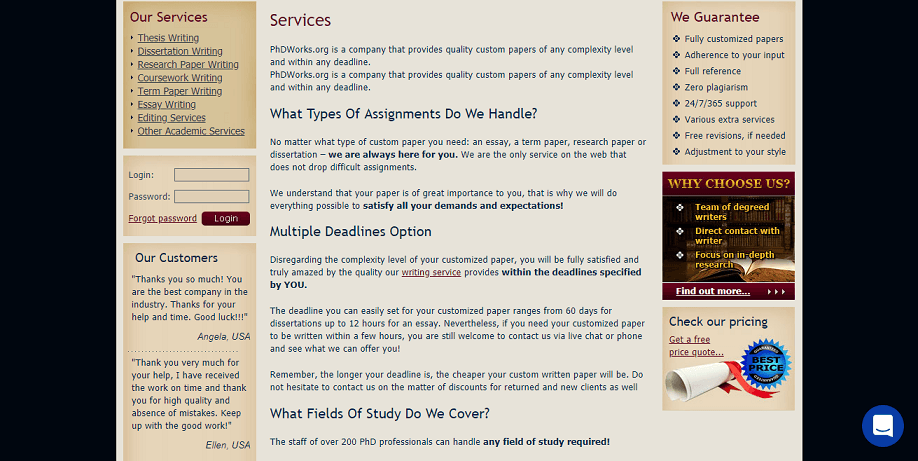The image displays an edited screenshot of a website with the top and bottom sections cropped out. The remaining front page of the website is set against a wide black background, leaving substantial empty black space on either side. The website itself has a light tan background. 

In the top left corner, there is a brown box, followed by a smaller, darker tan box centrally placed below it. A larger tan box sits below the darker tan box. The central area of the website maintains the light tan background, contrasting with the surrounding boxes.

On the right side of the page, there is a prominent tan box titled "We Guarantee" at the top, containing a bulleted list detailing the company's guarantees. Below this, in the central-right panel, a small box labeled "Why Choose Us?" provides additional information. At the bottom-right, a very small box with the text "Check Our Pricing" offers navigation to pricing details.